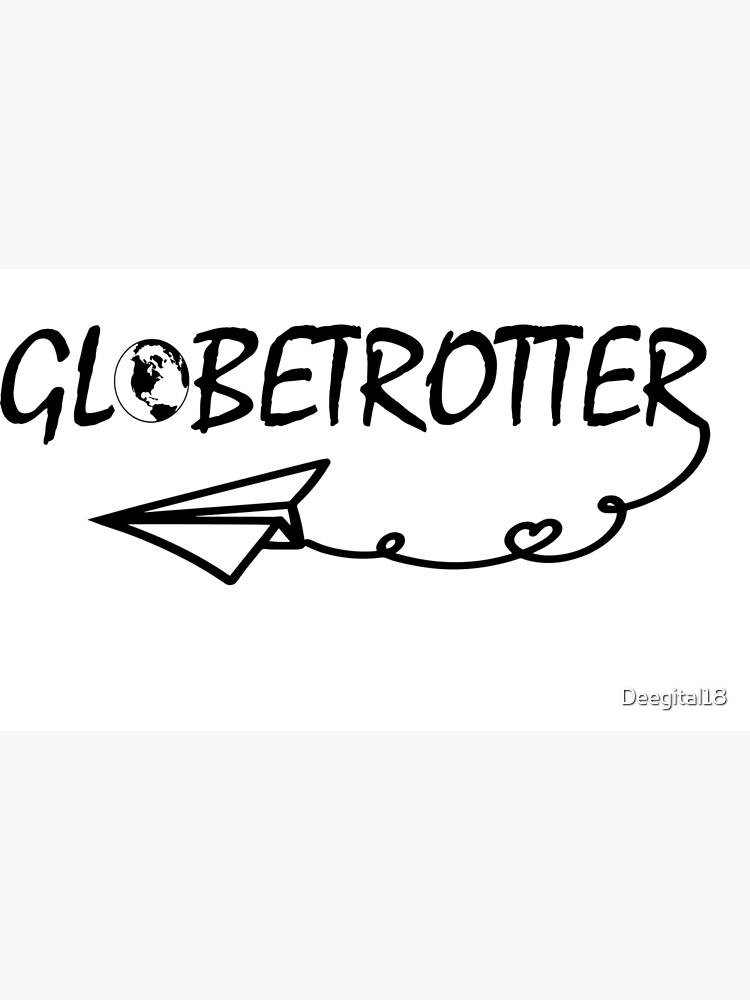The image is a vectorized black and white logo featuring a distinct scribbly, marker-style typography. The text reads "Globetrotter," with each letter thickly and irregularly drawn. The initial 'O' in "Globetrotter" is replaced by a globe icon, likely sourced from the Wingdings family, resembling the Earth with detailed continents. The background is predominantly white, with subtle gray shading at the top and bottom edges. Extending from the terminus of the 'R' in "Globetrotter" is a squiggly line, reminiscent of an old-fashioned telephone cord. This line curves and loops into a circling shape, culminating in a paper airplane aimed to the left, positioned beneath the globe icon. In the bottom right corner, there is a watermark with white text and a black drop shadow, which reads "DGTAL18".